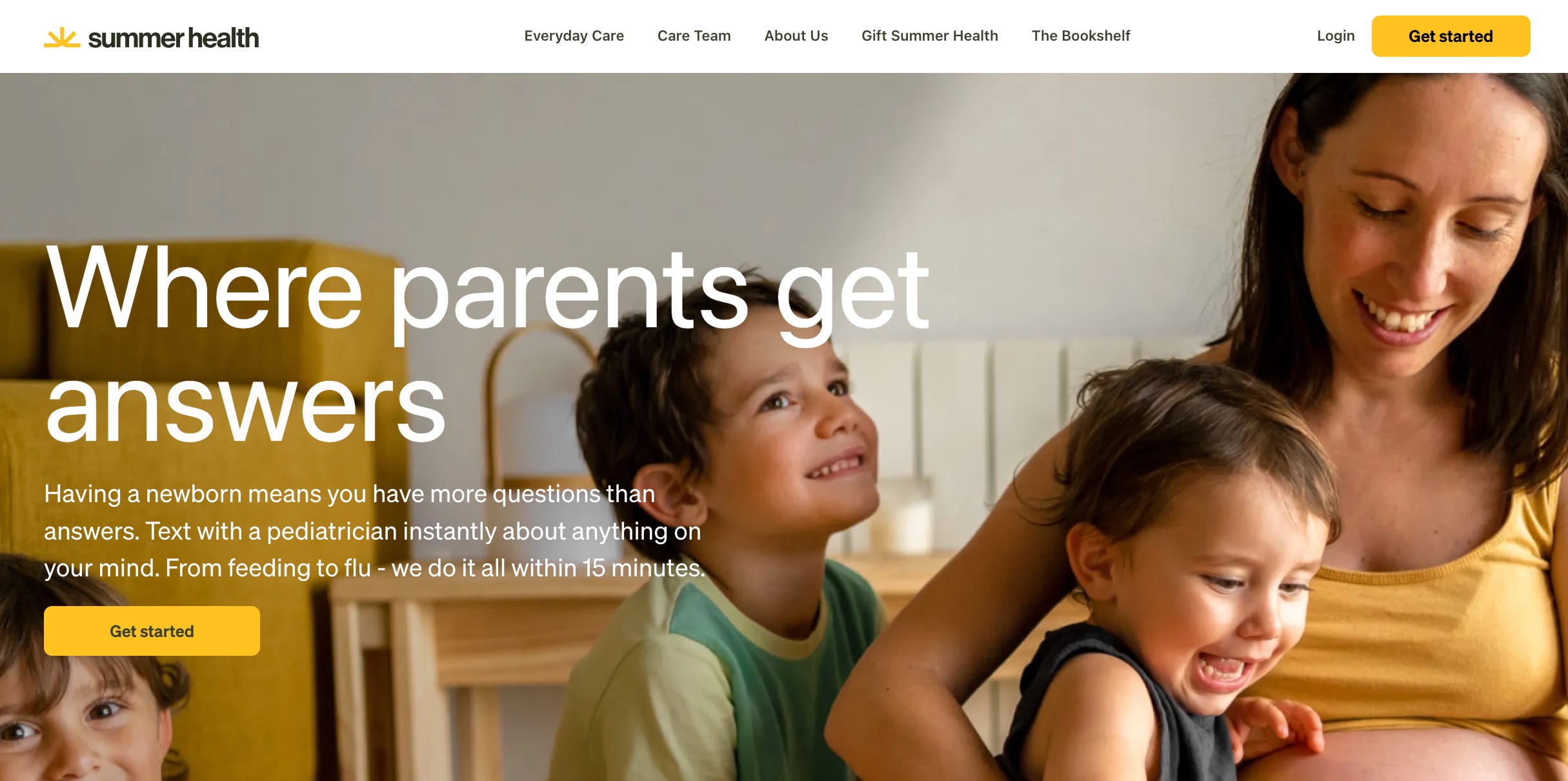**Image Description:**

The image showcases a web page titled "Summer Health." On the left side, there's a logo resembling a half sun in yellow, accompanied by the text "Summer Health" in bold black letters.

At the top center of the screen, there is a navigation menu with the following options in lighter, non-bold text: 
- "Everyday Care"
- "Care Team"
- "About Us"
- "Gift Summer Health"
- "The Bookshelf"

In the top-right corner, there is a login button next to a yellow button labeled "Get Started" in bold black text.

The central part of the image features a warm, inviting scene. A mother with brown hair is situated on the right, wearing a yellow shirt that reveals her pregnant belly. She is smiling, showing her front teeth, and holding a likely three-year-old child with brown hair and an open mouth, dressed in a gray tank top. Beside her arm is another smiling child, also with dark brown hair, wearing a green color-blocked shirt. In the bottom left-hand corner, there's another child with dark brown hair, but their face is partially cut off from the image.

Overlaying the image, bold white text states, "Where parents get answers." Below this, in lighter white text, it reads, "Having a newborn means you have more questions than answers. Text with a pediatrician instantly about anything on your mind. From feeding to flu, we do it all within 15 minutes." Beneath this text, there is a yellow button with black lettering that says, "Get Started."